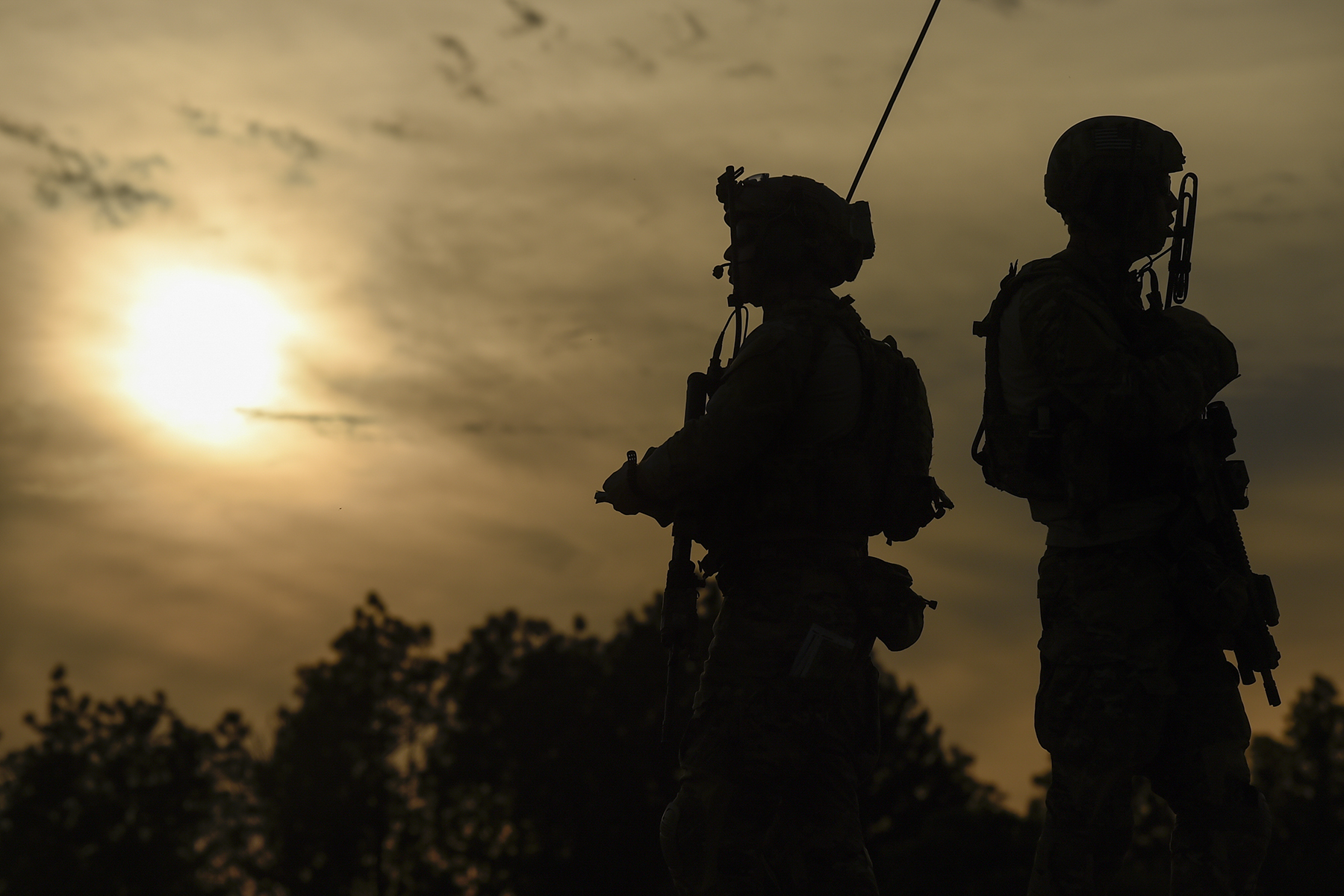A moody photograph taken at sunset or dusk, with a dramatic sepia tone filter, features a cloudy and overcast sky devoid of blue, with the sun barely peeking through the thick clouds. In the foreground, two silhouetted figures, presumably soldiers based on their tactical gear and helmets, stand back to back. The soldier on the right appears to be holding a gun while each faces opposite directions, to the left and the right. The distant silhouettes of trees add depth to the image, further enhancing the somber atmosphere. Predominantly dark and light browns dominate the color palette, lending a strong yet simple aesthetic to the photograph.